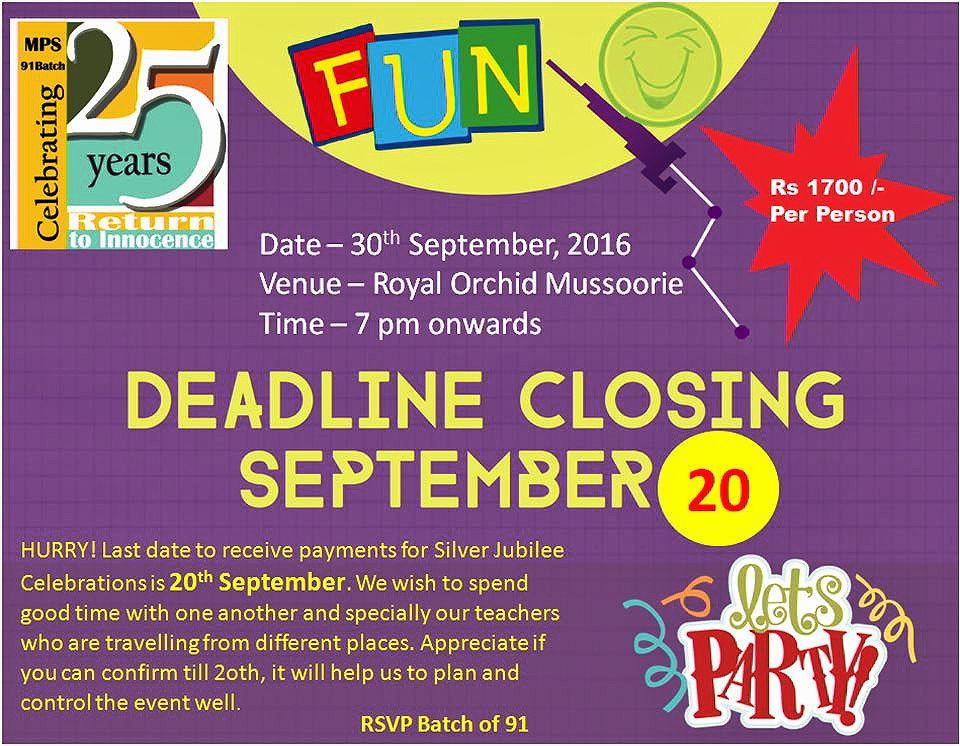The poster for the event is a vibrant and colorful flyer with a predominant purple checkered background, featuring an energetic and celebratory tone. At the top, large colorful block letters on a yellow background spell out "Fun!" along with a cheerful smiling face. To the left of the headline, there's a colorful logo proclaiming "Celebrating 25 Years: Return to Innocence" for the NPS 91 batch.

The details include:
- **Date**: September 30th, 2016
- **Venue**: Royal Orchid, Moosorée
- **Time**: 7 PM onwards
- **Entry Fee**: RS 1700 per person

Highlighted in various colors such as yellow, green, red, blue, and orange, the flyer emphasizes important information such as the deadline for payments, which is September 20th. It urges attendees to hurry, stating, "Last day to receive payments for Silver Jubilee celebrations is September 20th." 

The flyer emphasizes a strong desire to gather and spend quality time together, especially with teachers who will be traveling from various places. There is an appeal for confirmations by September 20th to aid in event planning and management. It ends with an enthusiastic "Let's party!" and a call to RSVP from the batch of 91. Colorful confetti graphics add to the festive spirit of the flyer.